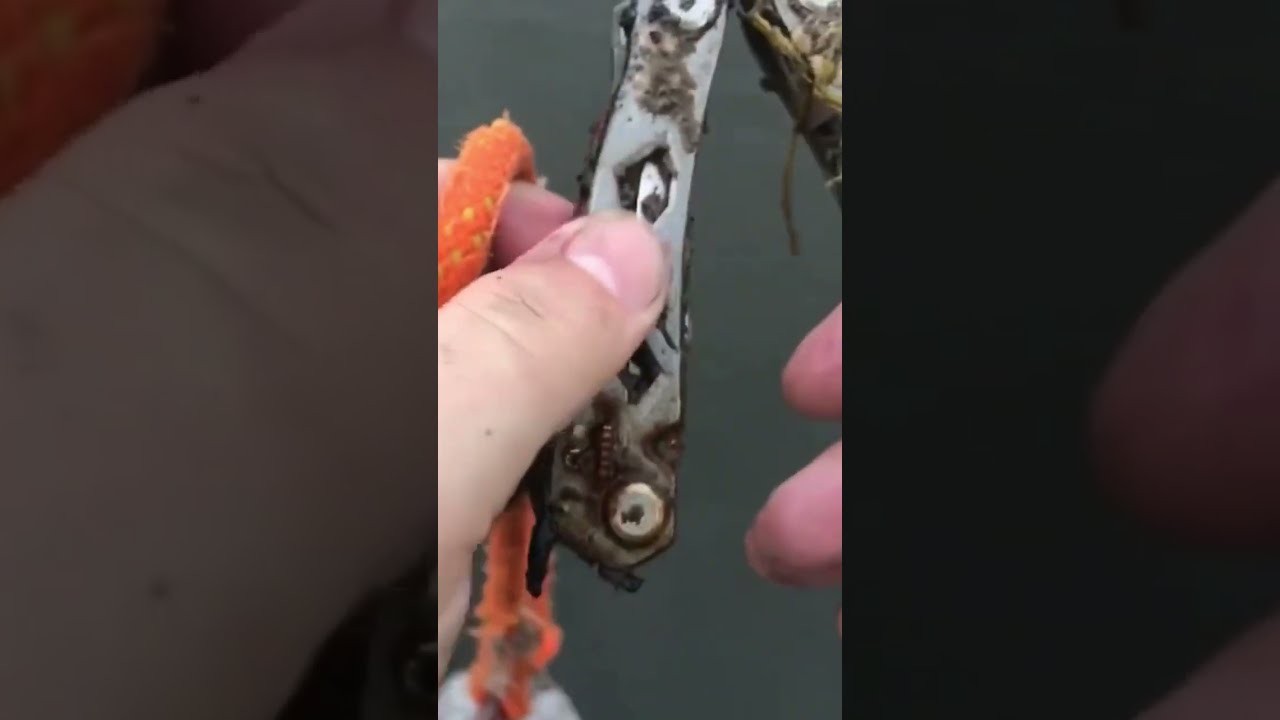A close-up image, seemingly a screen capture from a video, shows a person's left thumb and forefinger grasping a dirt-covered, silver switchblade knife. The tool appears relatively new but is muddied, possibly having been recently unearthed. An orange rope with yellow specks loops around the person's index finger, adding a splash of color to the scene. The knife, central in the frame, extends vertically with its blade pointing downward. The person's right hand, visible on the right side, touches the blade. The background, a blurred gray surface, hints at concrete. This intimate and detailed composition captures the interaction between the person and the items.